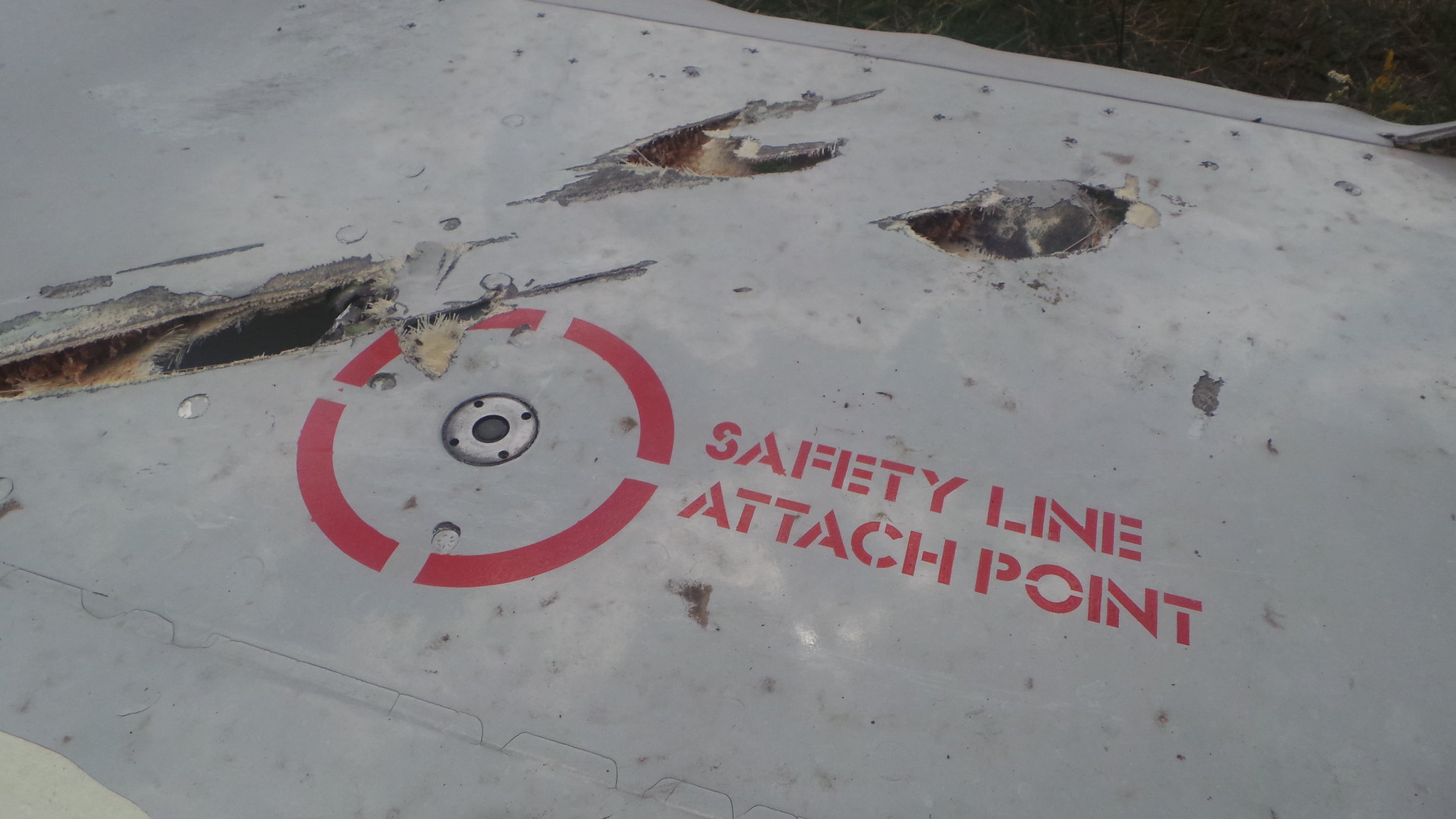This photograph captures a white fiberglass board, heavily damaged with multiple tears and puncture marks, that has fallen flat on the ground. The image is taken from an overhead angle, revealing the board's cracked surfaces and the stringy material connecting the broken parts. Prominently featured is a red circle with perforated lines located towards the center-left of the board. To the right of this circle, the text "SAFETY LINE ATTACH POINT" is written in bold red capital letters. Inside the perforated circle, a metal bracket is visible, featuring a black round receptacle presumably meant to secure a rope or similar attachment. The ground beneath the board is partially visible, showing patches of green grass, confirming the outdoor setting. A metal cap is seen at the top of the image, contributing to the metallic elements that underscore the board's battered state. The overall scene suggests a safety-related component that might typically be found at a workplace or industrial site.